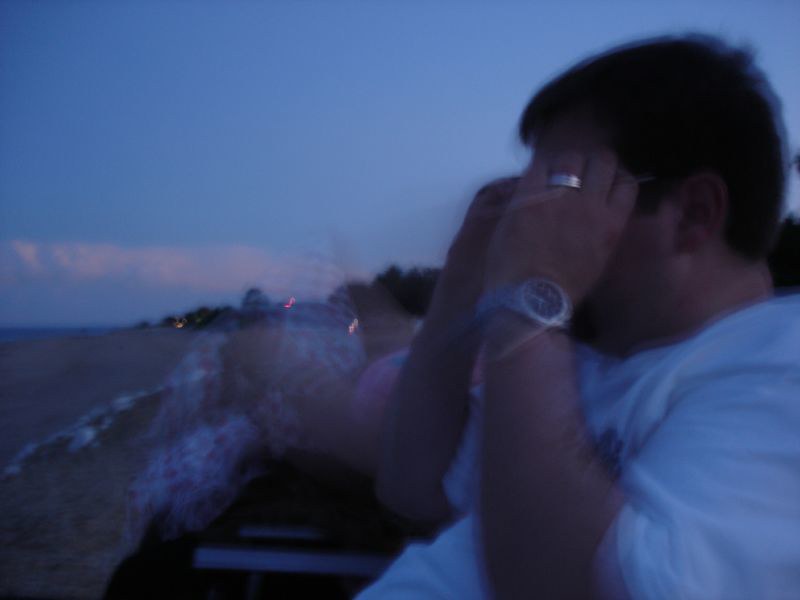In this outdoor close-up image, taken at what appears to be twilight or possibly under odd lighting conditions, a heavy-set man with short, dark hair, which may be slightly curly, is captured in a side profile view. His face is obscured as he holds both hands up to his eyes, possibly putting on or adjusting glasses. The man is wearing a white t-shirt, a silver or metallic chrome watch with a black face on his left wrist, and a wedding ring. 

The background is quite dark, suggesting it could be nighttime or dusk, with a dark blue sky. On the horizon to the left, there are a few houses with lights on and some trees visible. There is an open field, and the man could be sitting on a bleacher, watching an event, possibly a game, although no other people are visible. The overall setting is ambiguous, with some mentioning of the possibility of a beach given the sandy expanse and translucent white and light brown hues in the blurry background. The sky above is very blue with streaks of white clouds.